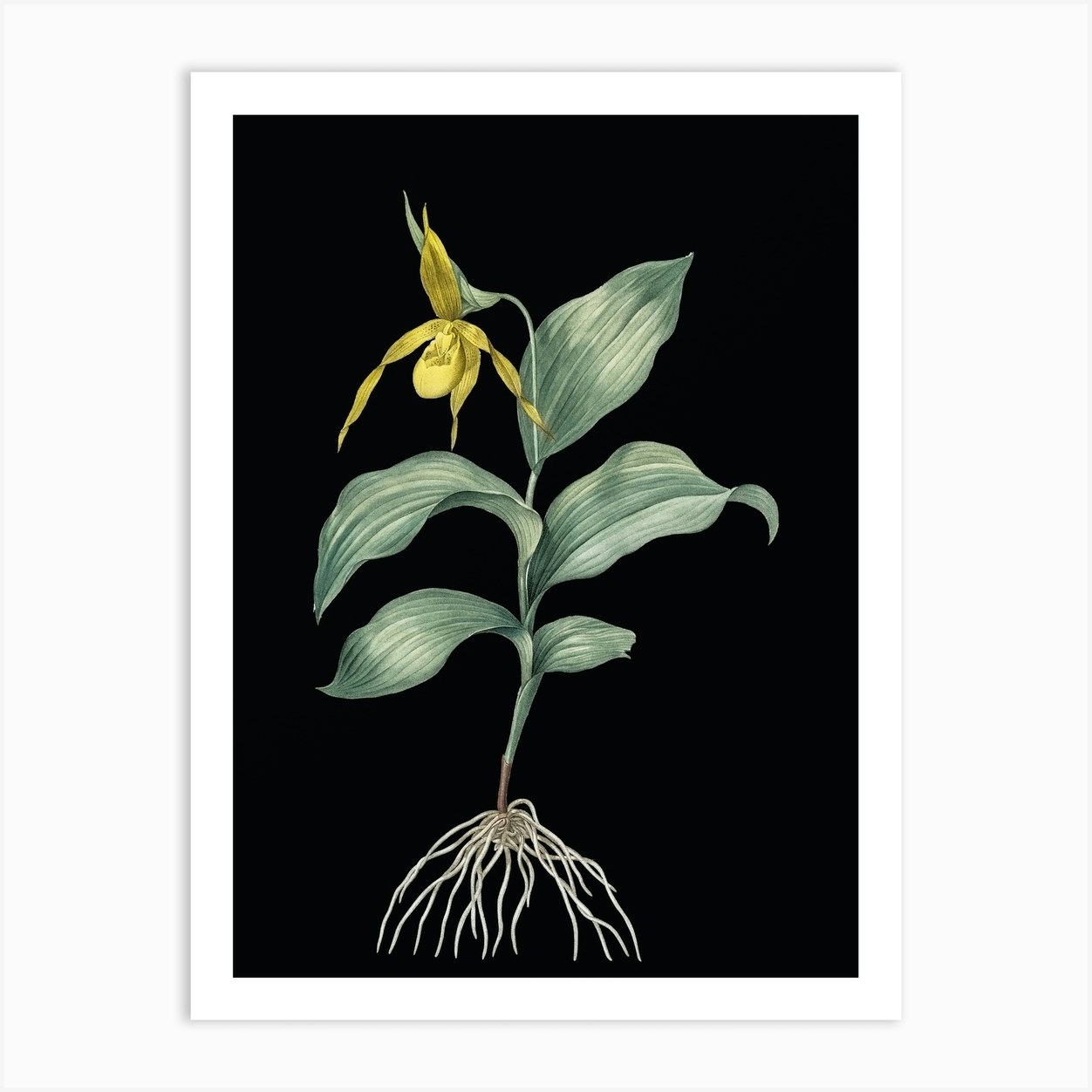The image displays a detailed, framed drawing of a plant, captured within several nested rectangles. The outermost layer is a very light gray rectangle, inside which sits a white rectangle with a shadow around it, giving the impression of depth. Within this white frame lies a black background that highlights the intricate design of the plant. This plant features six prominent, thick green leaves—three on each side—along a somewhat slender, brown stem. The stem extends upward to a yellow flower that appears to be wilting slightly, comprising seven petals and an oval-shaped center. Towards the bottom of the plant, there is a sprawling network of roots, depicted with numerous brownish-gray strands. The overall presentation of the artwork, with its striking black backdrop and detailed root structure, makes the depiction resemble a photograph at first glance, but closer inspection reveals it to be a carefully rendered drawing.